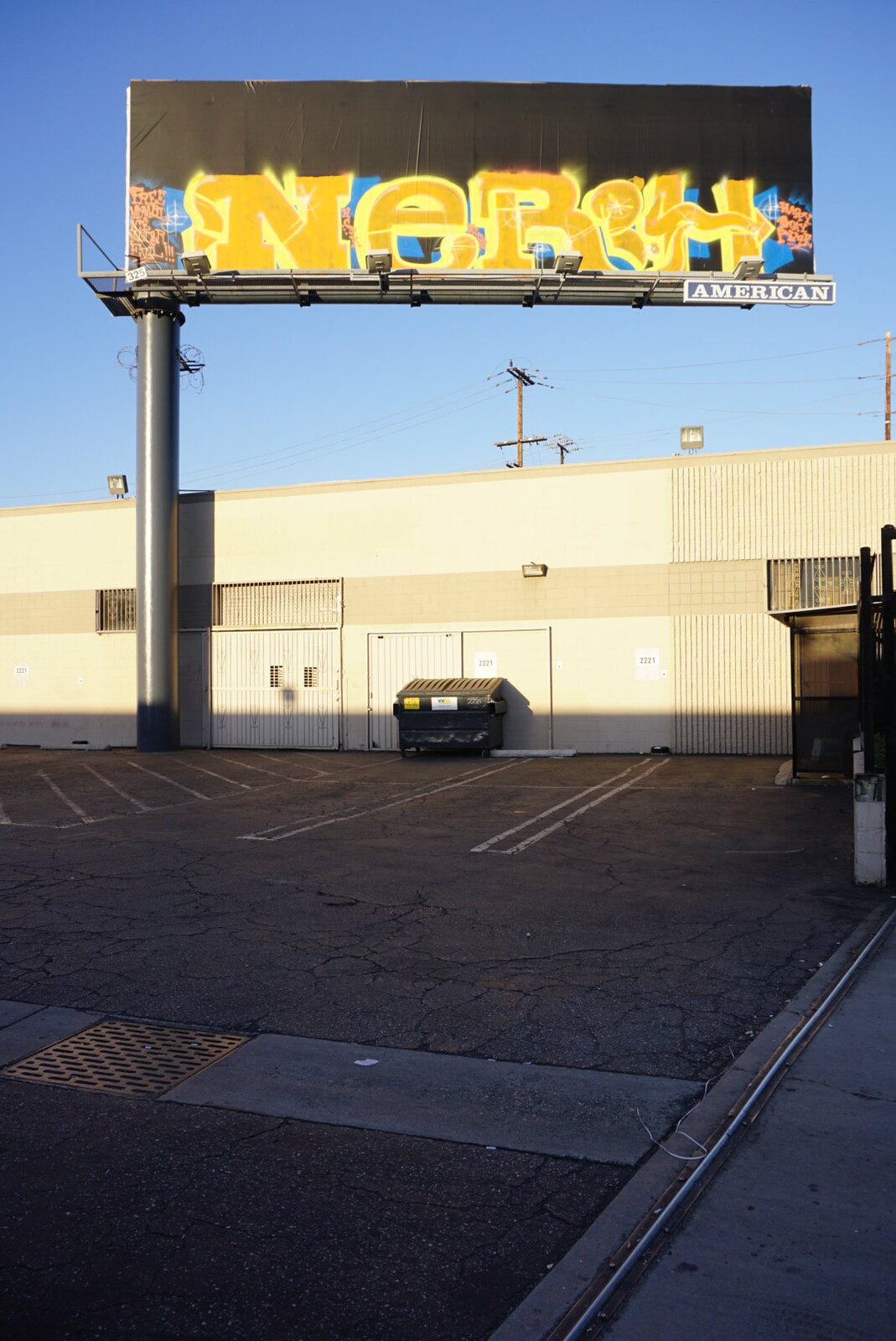In this vivid color photograph, we are observing a section of a parking lot under a blue sky. Dominating the upper portion of the image is a large rectangular sign, mounted on a sturdy metallic pole situated on the left. The sign features intricate yellow lettering, reading "N-E-O-R" and possibly another unreadable letter, followed by an ornamental "H," also outlined in yellow. The sign incorporates shades of blue and red, while the top edge appears black or shrouded in shadow.

Beneath the sign stands a tall beige wall adorned with a palleted design. Above the wall, power lines stretch horizontally, adding an industrial touch to the scene. In the center of the wall near its base is a dark rectangular object, adorned with an unreadable yellow label on the left and a white label in the middle.

The lower portion of the photograph reveals the parking lot itself, marked by white painted lines designating spaces. A metal grill is visible towards the lower left side, and a section of pavement rounds out the scene in the lower right-hand corner, contributing to the everyday urban aesthetic of the image.